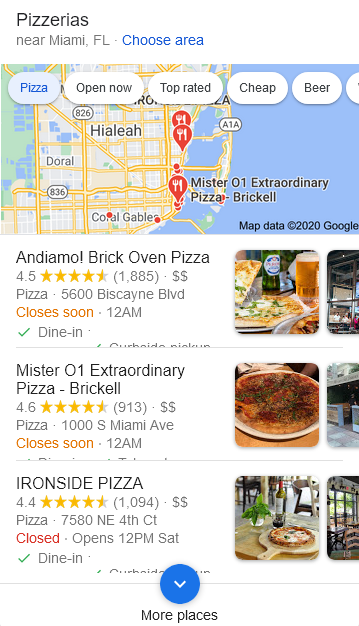This image depicts various locations of pizza establishments near Miami, Florida, categorized under "areas" and featuring options that are "open now" with a focus on affordability. These establishments include Mr. 01 Extraordinary Pizza, Pizzabrico in Doral, and Coral Gables. Additionally, the image highlights that some of these pizza places, such as Andiamo Brick Oven Pizza and Pizza 01 Extraordinary Pizza, have high ratings of 4.5 stars and 4.4 stars, respectively. According to the description, the first two listings are nearing their closing times, while the third one is currently closed.